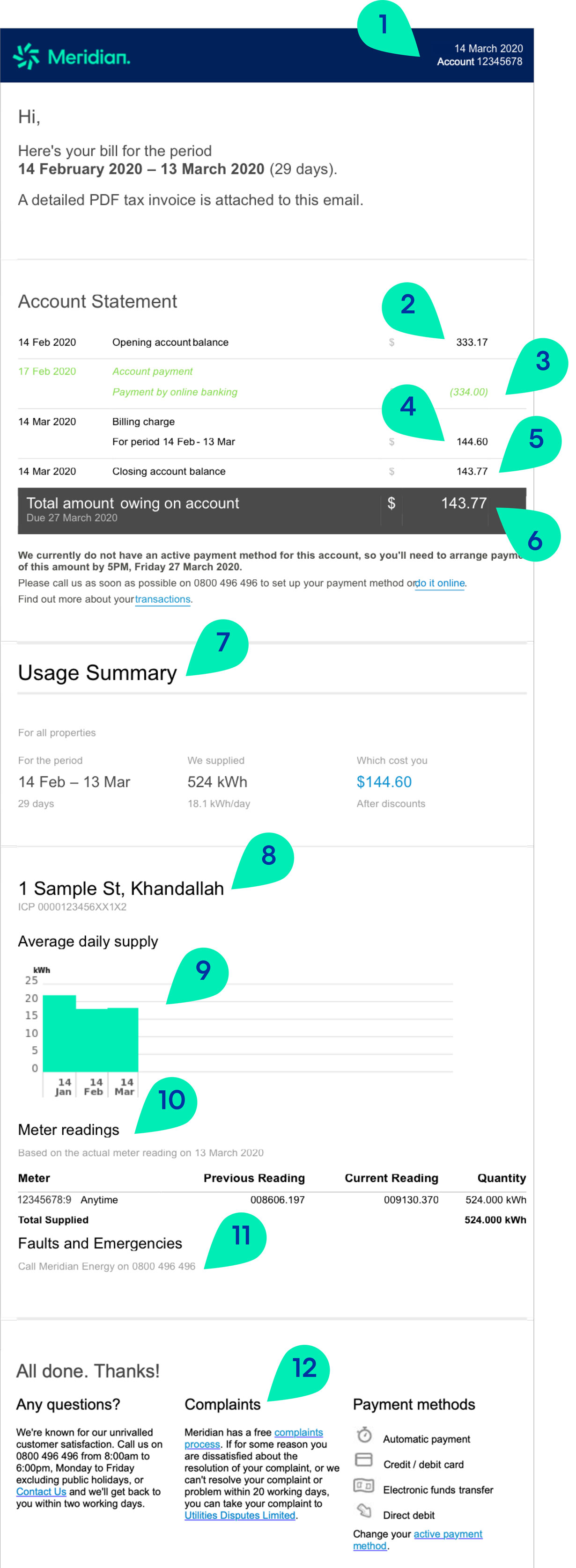Detailed Caption: 

"The image displays a notification from Meridian dated March 14, 2020, addressed to account number 12345678. It informs the recipient of their bill for the period from February 14, 2020, to March 13, 2020, covering 29 days. A detailed tax invoice in PDF format is attached to the accompanying email. The notification highlights that there is no active payment method associated with this account, urging the recipient to arrange for the payment by 5 p.m. on Friday, March 27, 2020. For setting up a payment method, the recipient is asked to call 0800 496 496 or complete the process online. The billing details include a usage summary indicating that 524 kilowatt-hours were supplied, costing $144.60 after discounts. The message concludes by inviting any questions and emphasizing the company's reputation for unparalleled customer satisfaction."